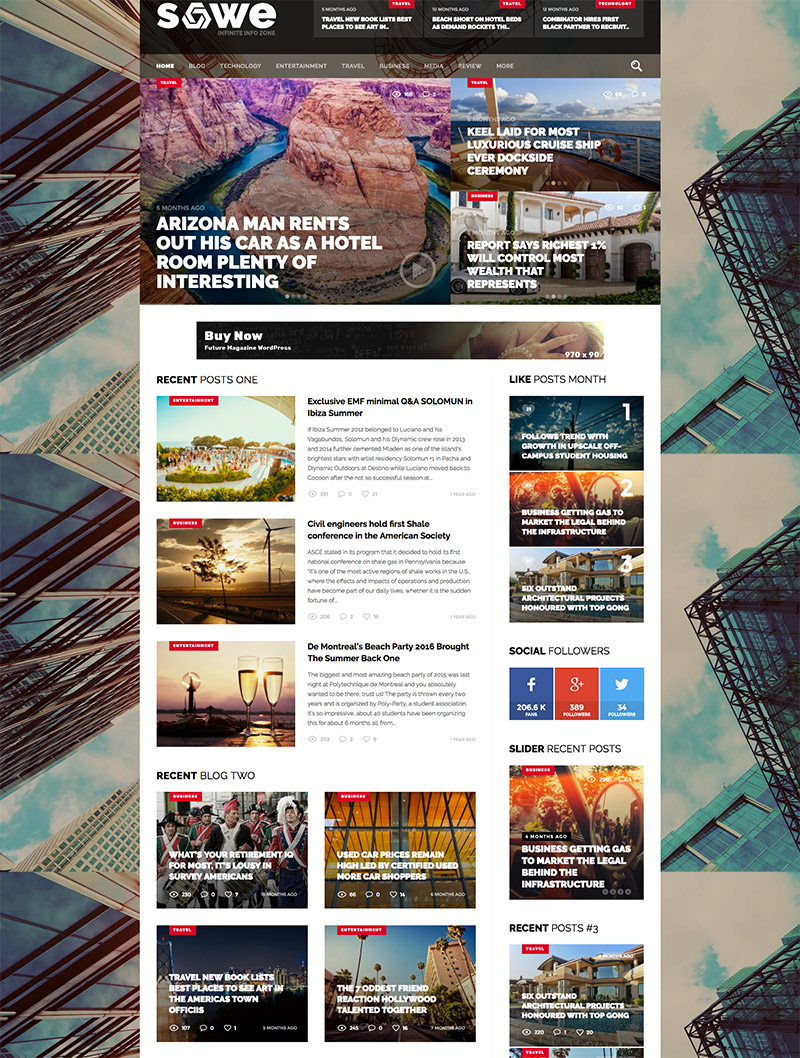**S.O.W.E. Website Interface Description**

At the top of the S.O.W.E. website, the name "S.O.W.E." is prominently displayed. Adjacent to the title are three tabs containing headlines, although the small text size makes them difficult to read. Below this header, there are navigation tabs, including Home, Blog, Technology, Entertainment, Travel, Media, More, Review, and a search icon.

The main content area is populated with various articles. The most significant article, occupying about a quarter of the page, features an intriguing story about an Arizona man who rents out his car as a hotel room. The image accompanying this article showcases a breathtaking mountain landscape in the background.

The page is vibrant with colorful stories and headlines scattered throughout. Centralized on the page are sections for recent posts, liked posts, and social media followings. At the page's bottom, additional stories, recent blogs, and posts are arranged into sliders marked as recent post one, recent post two, and recent post three. However, the small font size makes the titles hard to decipher.

Enhancing the visual appeal, the website's background features a repeating image of towering skyscrapers, providing a modern and urban aesthetic to the interface.